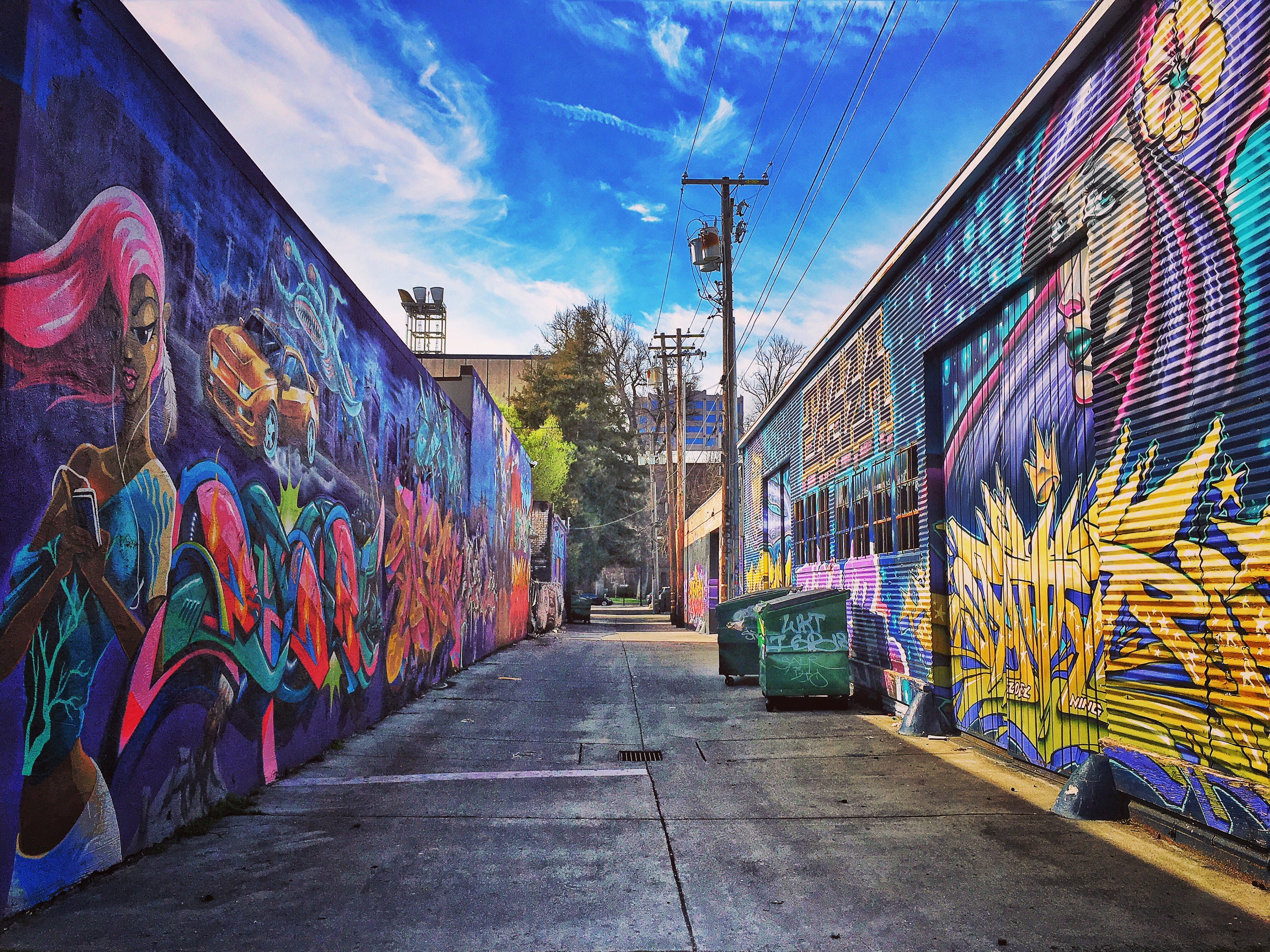This image captures a vibrant, clean alleyway set between industrial buildings, their walls exquisitely adorned with professional street art. On the left, a woman with pink hair, attired in a white crop top and shorts, is depicted texting on her phone, backed by a golden-yellow car. Her image is painted over a dark blue-indigo background. The opposite wall features a striking woman with purple and pink hair and a yellow hibiscus in her hair. She has blue lipstick and piercing blue eyes. Below her, a gold graffiti signature with a crown stands out. Additional graffiti, filled with big, bold, and multicolored shapes and random designs, enhance the walls further down. Details of graffiti writing in yellows, blues, pinks, and purple hues are visible, although the text is indecipherable. The two green garbage dumpsters also bear graffiti. Utility poles, one supporting a transformer, and a tree are present. Above, a clear blue sky with wispy, white clouds adds to the brightness of the scene.